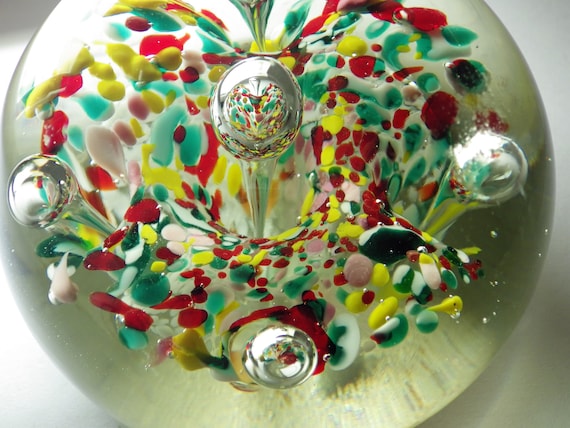This close-up photo captures a nearly spherical glass-blown object with intricate, abstract designs. The object, reminiscent of a marble or decorative art piece, is set against a completely white background, which enhances its vivid colors and clear structure. The top, bottom, and parts of the right side of the sphere are cut off due to the tight framing of the image. 

Within the clear glass, there's an array of colored patterns featuring hues of yellow, red, green, and hints of pink and white. These colors form bubble-like blobs suspended inside, creating an artistic, fiery blend. Additionally, there are four noticeable internal bubbles, possibly with pointed ends, resembling spikes or water drops. Scattered throughout the clear glass are small, delicate bubbles that add texture and depth to the appearance. The white surface the object rests on casts soft shadows in the upper left and lower right corners, further defining its dimensional form.